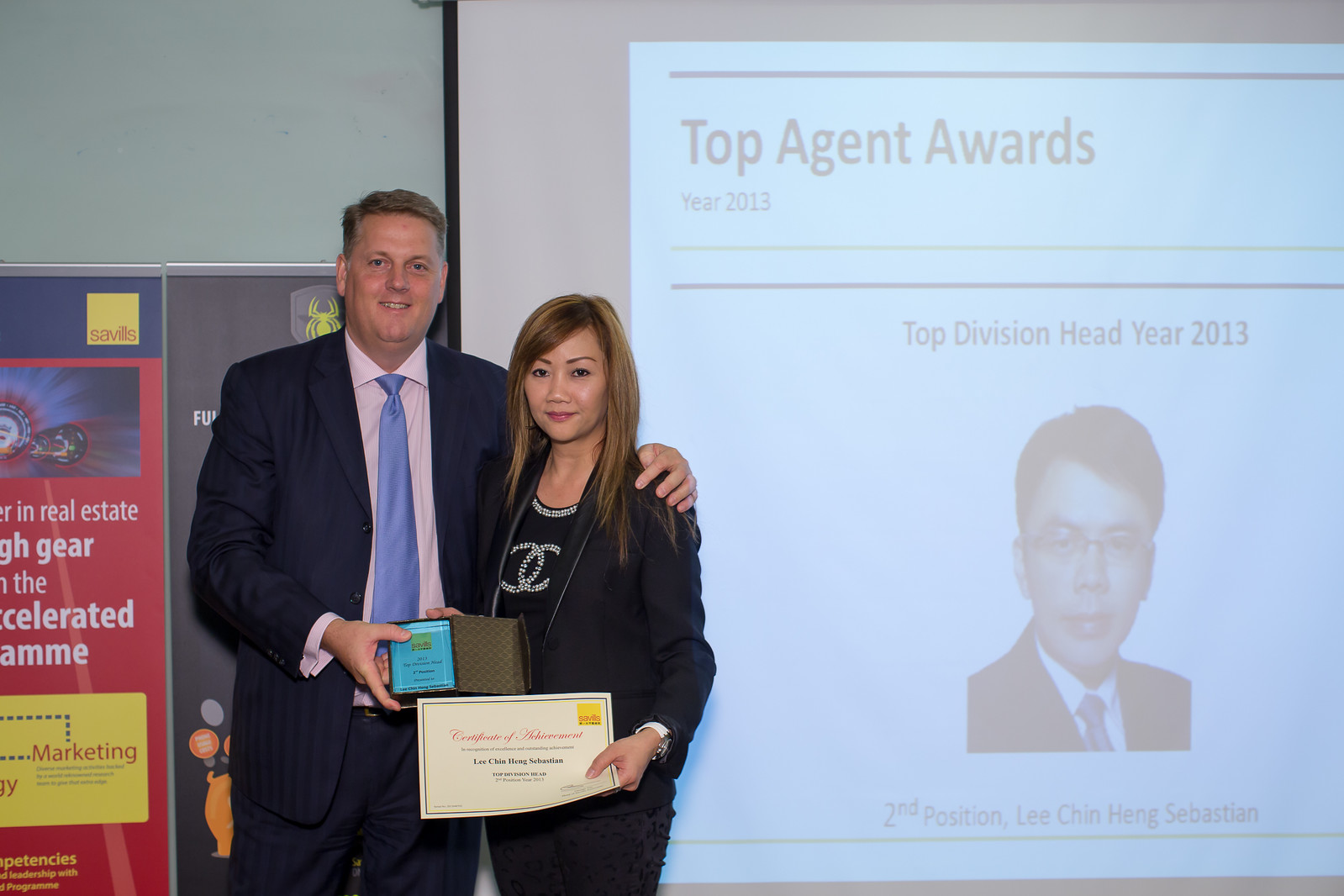The image depicts a celebratory moment during the Top Agent Awards Year 2013 ceremony. At the center, a woman with brown hair, dressed in a black suit and blouse, is receiving an award. In her left hand, she holds a white certificate, while her right-hand side companion, presumably the director or boss, stands with his left arm comfortably draped over her shoulder. The man is dressed in a coordinating blue suit with a light blue tie and a white shirt, and he smiles warmly, holding a blue-fronted box. Behind them, a projected screen displays the text "Top Agent Awards Year 2013" and "Top Division Head Year for 2013," along with an image of Lee Chin Heng Sebastian, labeled "Second Position." Additional elements in the background include banner advertisements, one prominently red and white reading "Real Estate Gear and Accelerated," suggesting a real estate context for the awards.